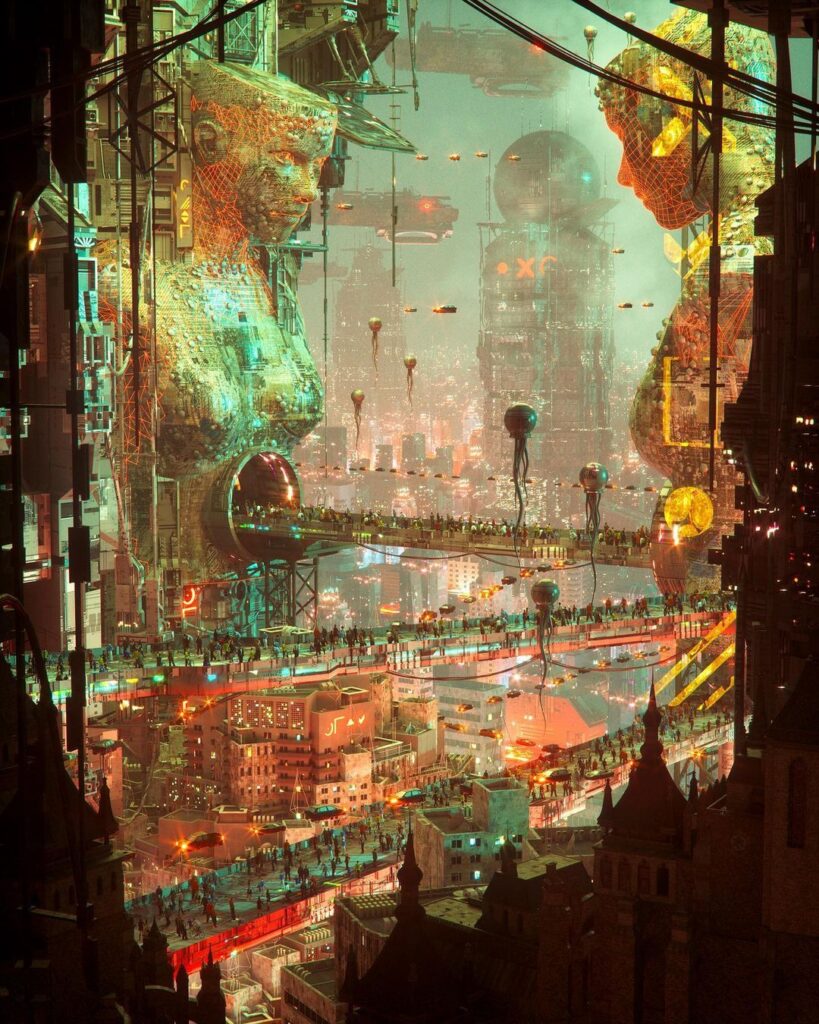This stunning piece of art, appearing as a surreal, dystopian poster or concept art for a futuristic city, features an extremely dense and vividly detailed urban landscape. Central to the composition is a busy city scene, where a multitude of people walks along streets and suspended walkways, weaving through an intricate tapestry of buildings and transport systems. Dominating the scene are two enormous statues of women, each several hundred feet high with gold and green faceted adornments, creating an overarching tunnel through their midsections. To the right, one of these statues stands prominently with her chest area and profile visible. Above these statues, a bridge teems with hundreds of pedestrians crossing between the massive structures. In the backdrop, a towering megastructure with a colossal spherical top looms large above the city, supported by rounded bases and draped with cables. Adding to the surreal atmosphere, floating alien-like creatures with tentacle-like tendrils drift through the air, while futuristic vehicles glide along aerial highways. Amidst the urban expanse, buildings range from traditional styles with spired rooftops and brick facades to modern and industrial designs. Dark shades of yellows, blues, and reds blend together, encapsulating the moody, dystopian essence of the scene, punctuated by glowing red lights from enormous spacecraft that hover high above the horizon.